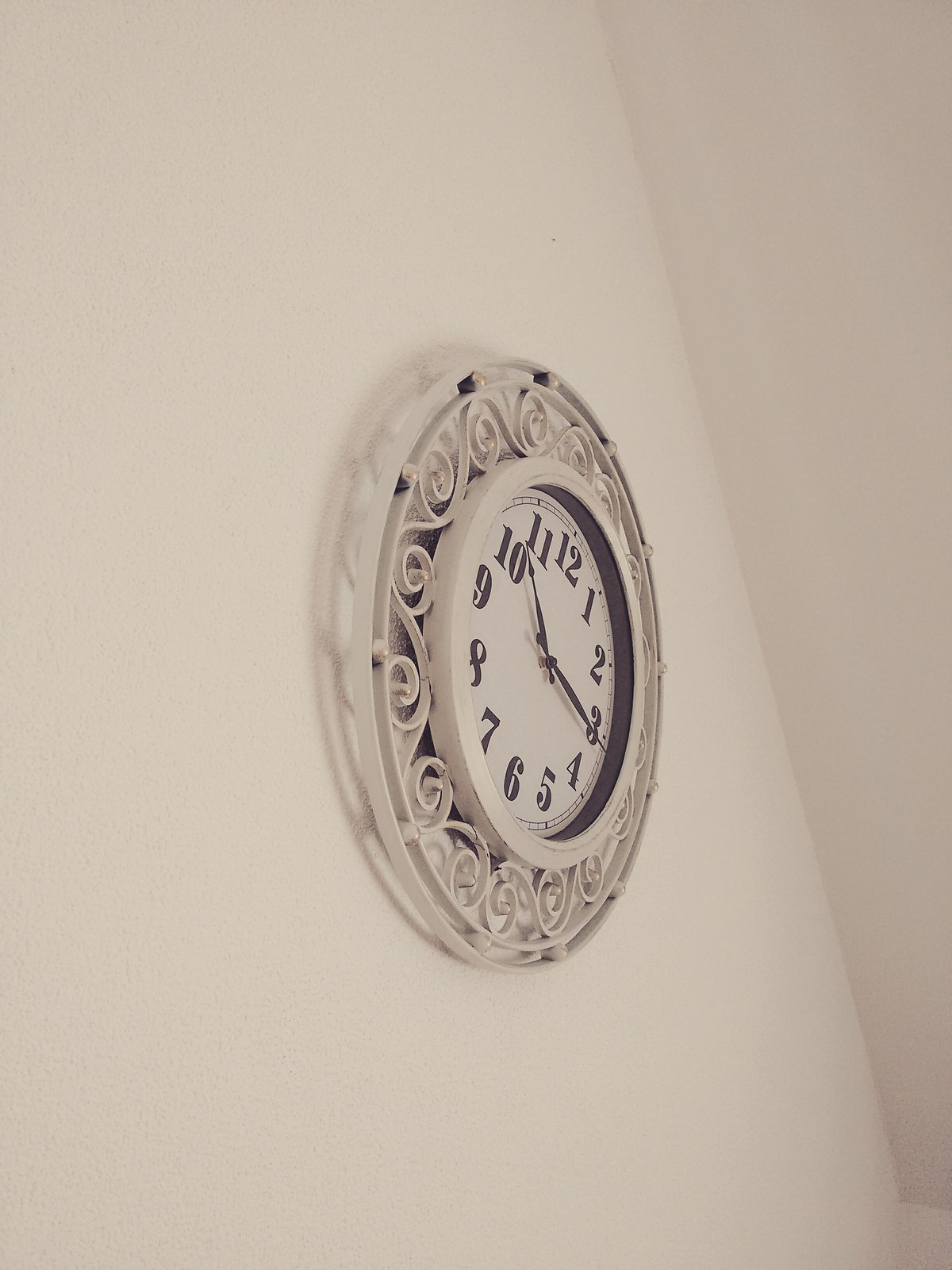This photograph showcases a decorative metallic wall clock with an intricate design. The clock is surrounded by a white bar, adding a clean, bright border to the piece. Encircling the clock is a beautiful swirl pattern, with each delicate swirl interlocking to form a complete, cohesive ring. This ornate design occupies a significant portion of the clock's outer area, creating an eye-catching frame for the smaller, central clock face.

The inner clock face, encased in glass, features large black numerals ranging from 1 to 12, with smaller dots or lines marking the individual minutes between each hour. The clock hands, also in black, consist of a minute and hour hand, with no visible second hand. The contrast of the black elements against the white background enhances the readability of the time while maintaining a minimalist aesthetic.

The photograph is taken from a lower left angle, providing a unique perspective of the clock's design and dimensions. The combination of the detailed outer swirl design and the clean, functional inner clock face makes this piece both a practical timekeeping device and an artful addition to any wall.